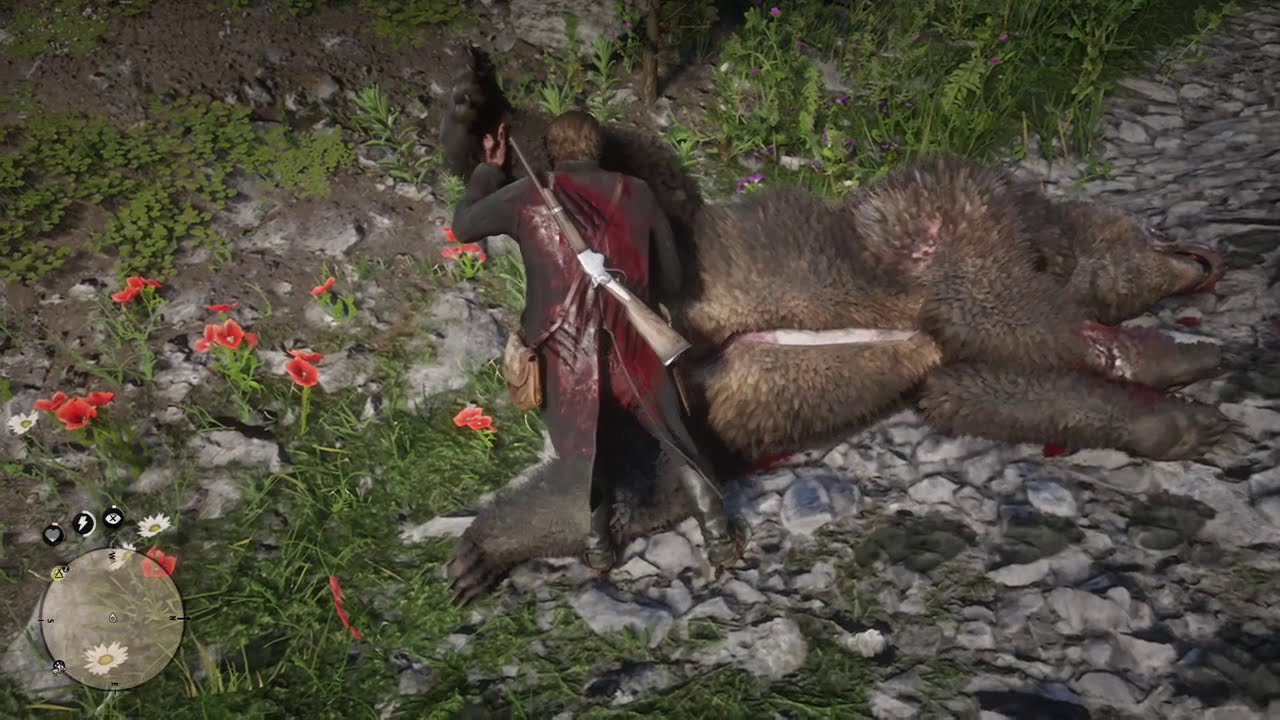The image, a high-quality video game snapshot, features a dramatic scene centered around a man wearing a long black duster coat, which is heavily stained with blood, particularly on his back. This character has brown hair and appears to be of middle age. Slinging a shotgun with a wooden stock and metal barrel over his back, the man stands in the middle of the image examining a dead black bear lying on a pile of rocks. The bear has a gruesome cut running up its stomach, with blood pooling underneath it. The scene suggests a recent fierce battle between the man and the bear, evident from the bear scratches on the man's back and the bear's exposed wounds. 

To the left of the dead bear, there are vivid pink and red flowers, contrasting with the surrounding green grass and scattered rocks, creating a wild, untamed setting. Additionally, a small trail bordered by rocks meanders off to the right. In the bottom left corner of the image, a translucent circular map or radar overlay features typical video game icons, including some health indicators for the character. The lighting in the scene is focused near the center, gradually darkening towards the edges, suggesting an early morning or late evening timeframe.